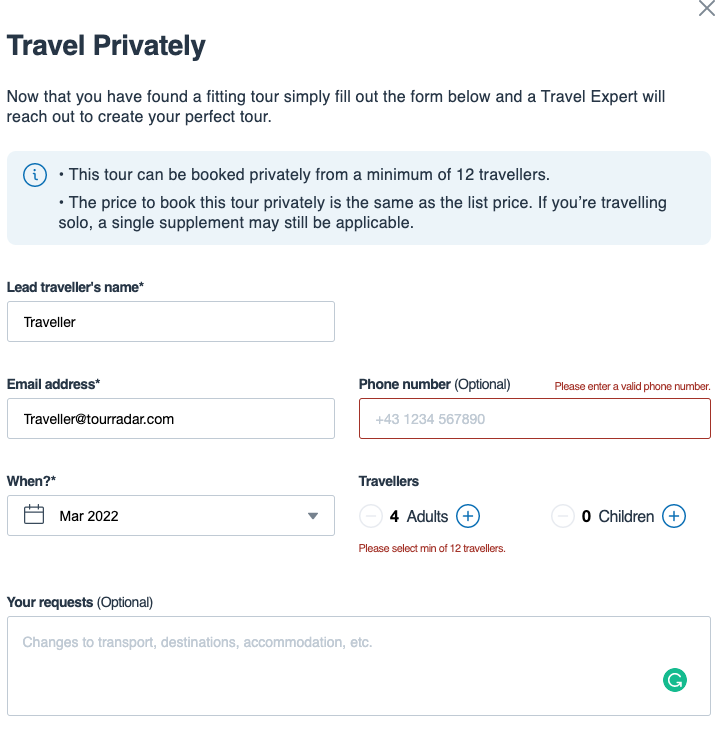Screenshot Description: 

The screenshot presents a web page with a clean white background dedicated to travel planning. Prominently displayed at the top is the headline "Travel Privately". Following the headline, there's informative text which reads: "Now that you have found a fitting tour, simply fill out the form below and a travel expert will reach out to create your perfect tour."

Below this, a blue rectangle with rounded corners houses a blue circle featuring an eye icon, accompanied by two bullet points which state: 
1. "This tour can be booked privately from a minimum of 12 travelers."
2. "The price to book this tour privately is the same as the list price."

A cautionary note follows, indicating that if you're traveling solo, a single supplement may be applicable.

The form begins with fields for user input:
1. "Lead Traveler's Name" labeled with an asterisk (*) indicating it is a required field.
2. "Traveler Email Address" also adorned with an asterisk, suggesting it's mandatory. Sample entries such as "traveler@tourradar.com" illustrate correct format.
3. "Phone Number (optional)" field is present, and above it, there is a red colored note stating "Please enter a valid phone number" indicating an error message.

Further down, there is a date selection field labeled "When?" with a question mark and an asterisk for required input, currently displaying "March 2022".

Lastly, there is a traveler count section denoted "Travelers", set to "4 adults". This field includes a user interface element with a circle featuring a plus sign (+) for adding travelers to the right, and a circle with a minus sign (-) for reducing the number of travelers to the left.